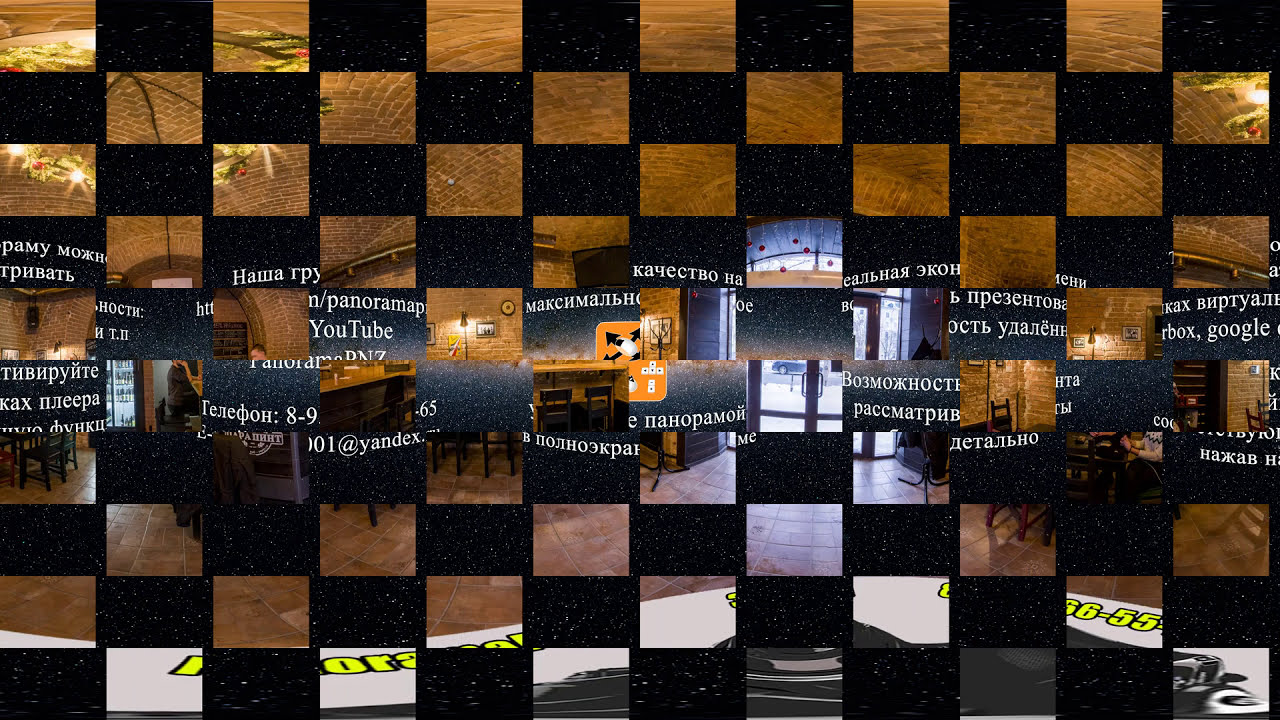The image features a perplexing checkerboard pattern, alternating between black and tan (or brown) squares. Intriguingly, some of the squares contain various images and text. In the center of the image, a doorway is visible amidst the checkered tiles, suggesting an indoor setting, possibly a dining area. Text in different languages, including what seems to be Greek, Cyrillic (possibly Russian), and English, runs across the squares. Legible words include "YouTube," "panorama," and "Google," while other text remains indistinct due to the checkerboard obscuration. Neon green block letters appear along the bottom, partially hidden by the pattern. On the lower right corner, there is a figurine and the numbers "36-55." The overall scene feels like a collage, blending realistic and abstract elements into a somewhat enigmatic visual.